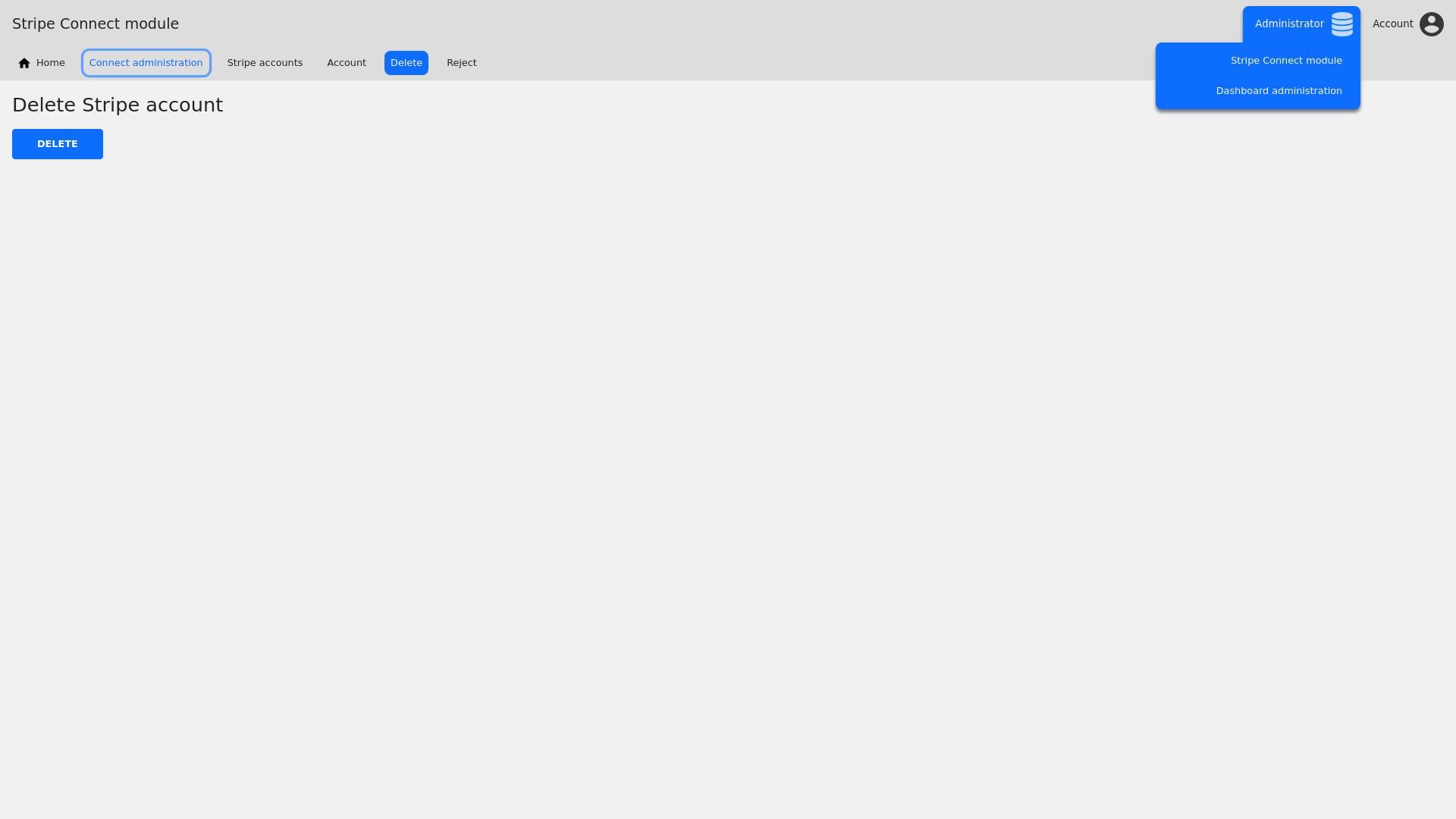This image is a screenshot displaying an interface set against a very pale gray background. The interface features a darker gray strip running horizontally across the top. In the upper left corner, "Stripe Connect Module" is displayed in black text. Directly beneath this, the text "Home" is located, followed by "Connect Administration" in blue text to the right. Subsequent options include "Stripe Accounts," "Account," and "Delete," with "Delete" highlighted in blue. At the far right of the darker strip, there is a blue background button labeled "Reject" in light blue text. Additionally, the text "Administrator, Stripe Connect Module, Dashboard Administration" is visible in light blue. In the upper right corner of the image, the word "Account" is followed by a standard dark gray icon depicting a human head and upper body.